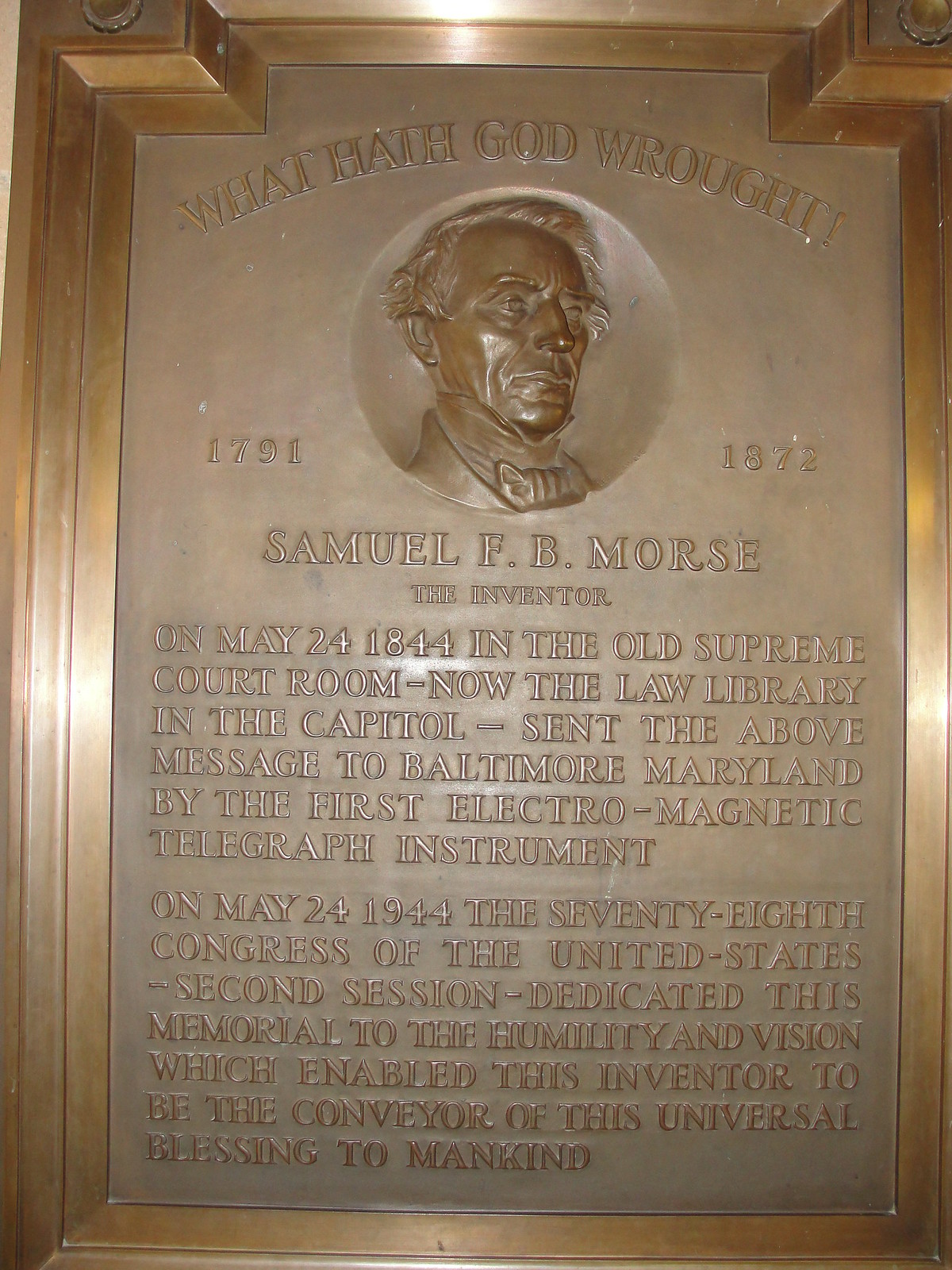This detailed and elegant metal plaque, possibly made of bronze, commemorates the life and achievements of Samuel F. B. Morse, a notable inventor. The plaque, which has a debossed image of Morse’s face, prominently features the inscription "What hath God wrought?" along with his lifespan dates, 1791 to 1872. The text explains that on May 24, 1844, in the Old Supreme Courtroom (now the Law Library in the Capitol), Morse sent the historic first message using the electromagnetic telegraph to Baltimore, Maryland. In honor of this milestone, and recognizing Morse’s humility and vision, the 78th Congress of the United States dedicated this memorial during its second session on May 24, 1944. The intricate carvings and historical notations suggest that this plaque is a significant piece, likely to be found in a museum or an esteemed institution, possibly a science museum.